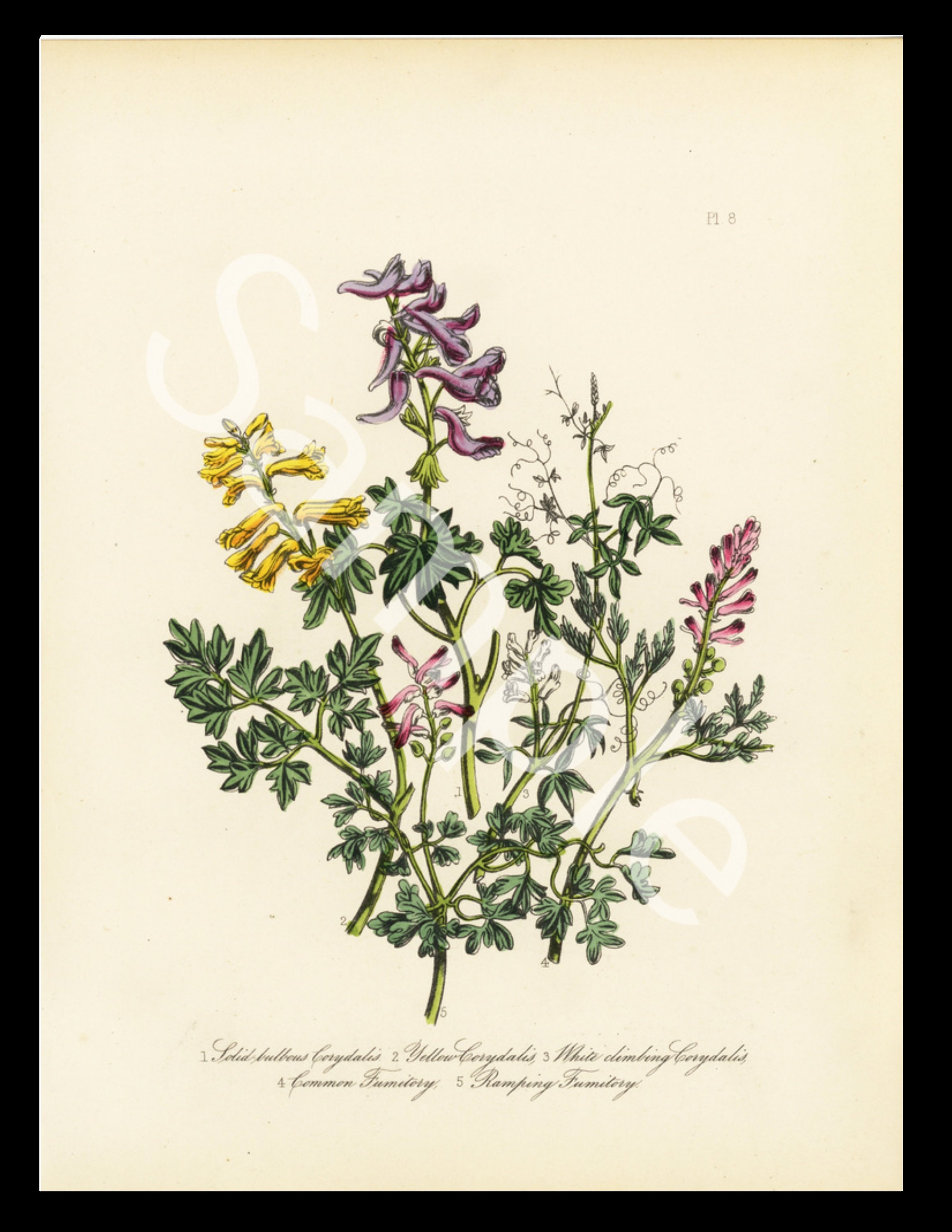The image is a vertically oriented, hand-painted artwork featuring a botanical subject, likely sourced from the internet as indicated by the translucent white watermark reading "sample" diagonally across it. It is encased in a narrow black border approximately a quarter-inch wide, set against an off-white to champagne-colored paper background that conveys an aged aesthetic. The central image depicts a detailed arrangement of plants with dark brown, almost dull green, four-tipped leaves and lighter green stalks. The flowers are varied: on the left, there are elongated yellow blooms; in the middle, purple fluted flowers; and to the right, smaller blooms with dark pink petals, some exhibiting dark purple tips. The composition also features delicate, swirly vine tendrils emerging from the foliage. Beneath the botanical illustration, there is cursive lettering and numeric labeling (1 to 5) suggestive of botanical taxonomy, although the specific words are indistinguishable.